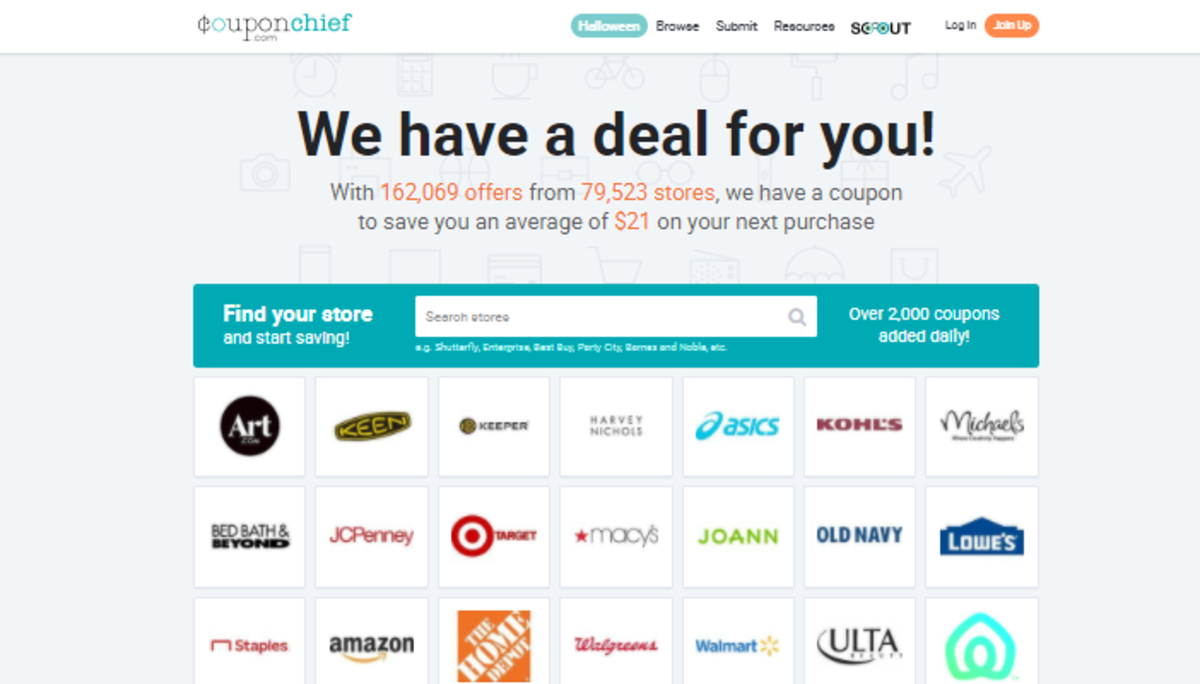In the image, we see a detailed screenshot of the Coupon Chief website. The very top of the page features a white border, with the website's name, "Coupon Chief," positioned towards the left side. On the right side of the top-most section, there’s a navigation menu which includes options such as "Halloween," "Browse," "Submit," "Resources," and a logo labeled "Scout." Adjacent to this logo, there is black text that reads "Log In," and beside it, an orange button with white text that likely says "Join Up."

Beneath this top section, the website sports a light gray background decorated with faint, outlined images of various items such as a clock, a cup, a bicycle, a keyboard, a mouse, a paintbrush, a paint roller, musical notes, and an airplane.

At the top of the main content area, there is a prominent heading in black text stating, "We have a deal for you." Below this heading, a subheading informs visitors in dark gray text (with specific numbers highlighted in orange) that they can find "162,069 offers from 79,523 stores" and save an average of "$21" on their next purchase.

Below this informative section lies a turquoise-bordered rectangular box containing a search bar. The search bar features black placeholder text that reads "Search store" with a magnifying glass icon to its right. To the left of the search bar, white text declares "Find your store and start saving." On the right side of the search box, white text indicates that "Over 2,000 coupons are added daily." Beneath the search bar, there appears to be small text that is unreadable at the current size.

Further down, the page displays a grid of white squares organized into three rows with roughly seven squares per row. Each square showcases the logo of a different brand or store. The first row includes brands and stores such as Art, Keen, Keeper, Harvey Nichols, Basics, Kohl's, and Michaels. The second row features Bed Bath & Beyond, JC Penney, Target, Macy's, Joanne Fabrics, Old Navy, and Lowe's. Lastly, the third row highlights Staples, Amazon, The Home Depot, Walgreens, Walmart, Ulta, and another brand with a distinctive logo involving a combined square and circle shape outlined in greenish-blue, with an inner curve forming an additional circle. Each of these brand names is written using the official logos of the respective companies.